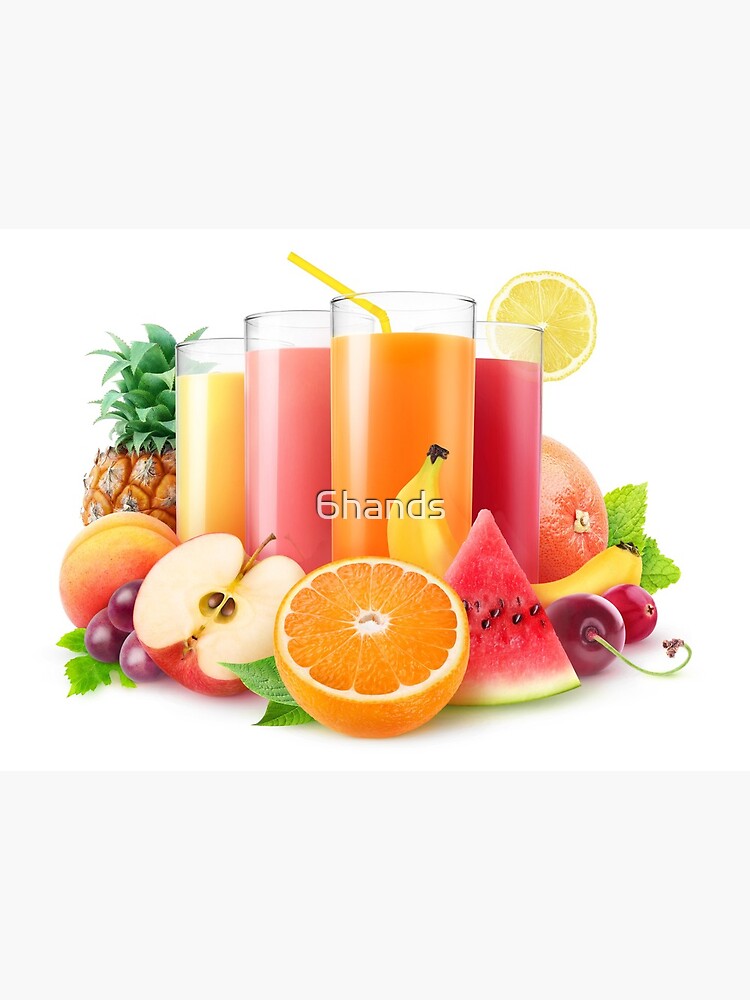The image presents a vibrant and enticing advertisement for a smoothie or pressed juice bar, perfectly suited for the back of a magazine. Centered in the image are four tall, thin, transparent glasses, each filled with a different color liquid: yellow, pink, orange, and a dark plum-red. The yellow smoothie is placed on the left, followed counterclockwise by a pink smoothie, an orange one with a yellow straw, and finally a dark plum-red drink garnished with a lemon slice. Surrounding the glasses is an abundant display of fresh fruits, including a whole pineapple, a peach, purple grapes, a halved apple, a sliced orange, a banana, a watermelon wedge with seeds, a grapefruit, mint leaves, and a cherry or red grape. The composition rests on a clean white background, with the text "Six Hands" prominently displayed in the middle, suggesting the artisanal quality of the drinks. The overall scene exudes freshness and deliciousness, appealing to health-conscious consumers.